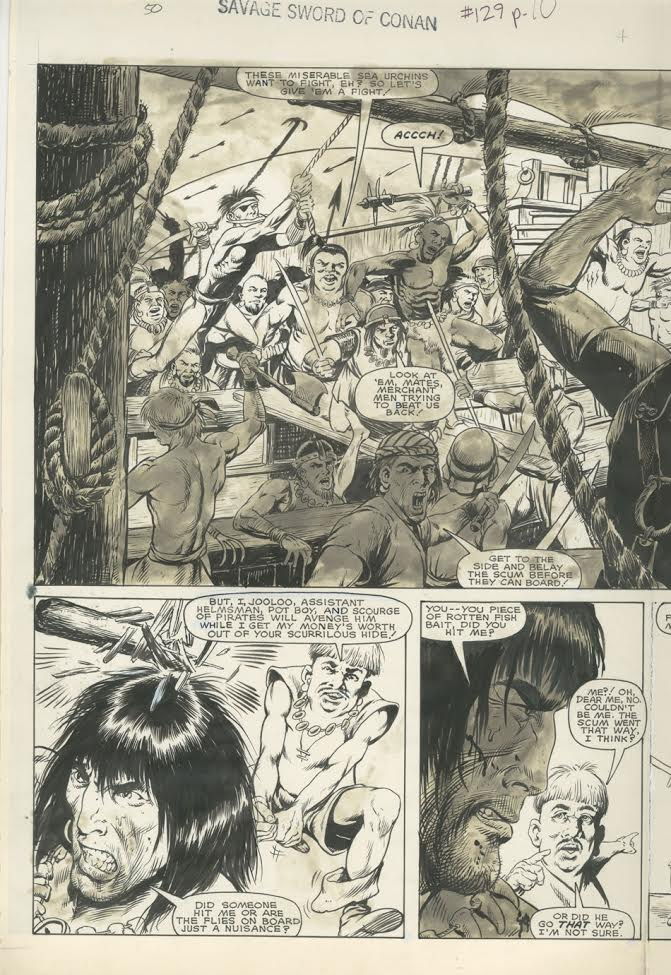The image depicts a page from the comic book "Savage Sword of Conan," specifically issue number 129, page 10. The page is drawn in black and white and consists of three main panels. 

In the top panel, there's a chaotic scene of what appears to be a mutiny or ship invasion on an old-time sailing vessel. The panel is bustling with action, as many bare-chested men wielding swords, axes, and spears are engaged in combat. Some men are seen climbing ropes to board the ship, with arrows flying through the air. A man wearing an eye patch stands out amidst the fray, and there are apparent Native American warriors among the attackers. The text in this section includes phrases like "These miserable sea urchins want to fight, eh? So let's give them a fight," and "Get to the side and repel the scum before they can board."

The middle panel, located below the chaotic battle, features a dramatic moment where a man strikes another over the head with a wooden club, causing it to break. The victim, possibly Conan, shows a mixture of anger and confusion, questioning aloud if someone hit him or if the sensation is just from flies on board. The assailant, a surprisingly fearful man, attempts to deflect blame.

The bottom right panel showcases the aftermath of the clubbing, with the injured man confronting his attacker. He angrily exclaims, "You piece of rotten fish bait. Did you hit me?" to which the assailant nervously denies involvement, directing blame elsewhere in a desperate attempt to avoid further conflict.